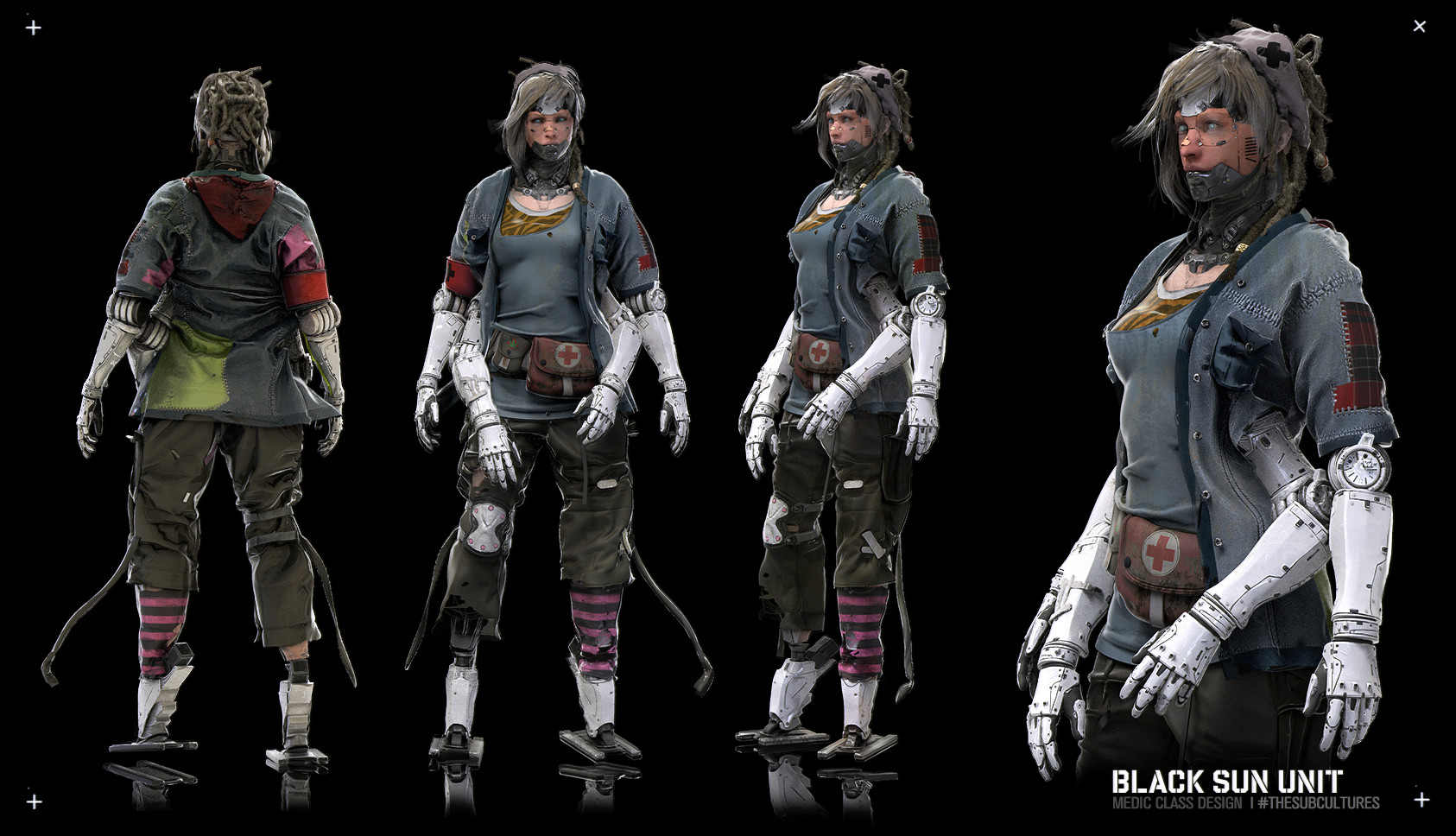The image is a detailed montage featuring an individual with a futuristic, robotic appearance, photographed in four different positions. The character resembles a post-apocalyptic warrior, reminiscent of Mad Max aesthetics. They have four mechanical arms, two on each side, with the extra set appearing to be robotic. The character, who has long brown hair and is presumably a white woman, is outfitted in a gray shirt and jacket. Their attire is complemented by dark brown pants rolled up to the knees, revealing metallic, robot-like legs and flat feet. The character's arms are covered in a metallic material, and one leg appears to be prosthetic. 

In the first image, they are seen from the back, looking away from the camera. The second image captures them facing the camera directly. The third image shows the individual at a two o'clock angle, looking to the right, a pose that is repeated in the fourth close-up shot, focusing from their upper legs to the top of their head. They wear a clear face mask, adding an extra layer of mystery to their appearance. 

A notable accessory is their belt, equipped with a fanny pack marked with a red cross, suggesting a medic role. The bottom right corner of the image contains the labels "Black Sun Unit" and "Medic Class Design, The Subcultures." This hints that the character may be from a video game or a fictional universe with distinctive subcultures.